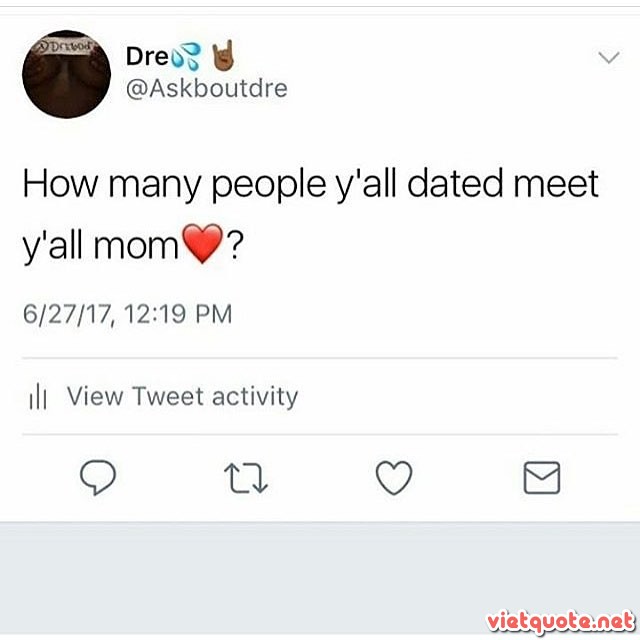This image is a screenshot of a tweet posted on June 27, 2017, at 12:19 PM by a user named Dre, whose handle is @ASKBOUTDRE. Dre's profile features two emojis next to his name: blue sweat droplets and a rock hand sign. His avatar seems to be a somewhat unclear or dark image, potentially depicting a person holding a sign. The tweet reads, "How many people y'all dated met y'all mom? ❤️?" Below this post, typical Twitter features are visible, including options to comment, share, and like, as well as a "View Tweet Activity" button. At the bottom right of the image, there is a watermark that reads "vietquote.net" in red text, with a gray border beneath it.